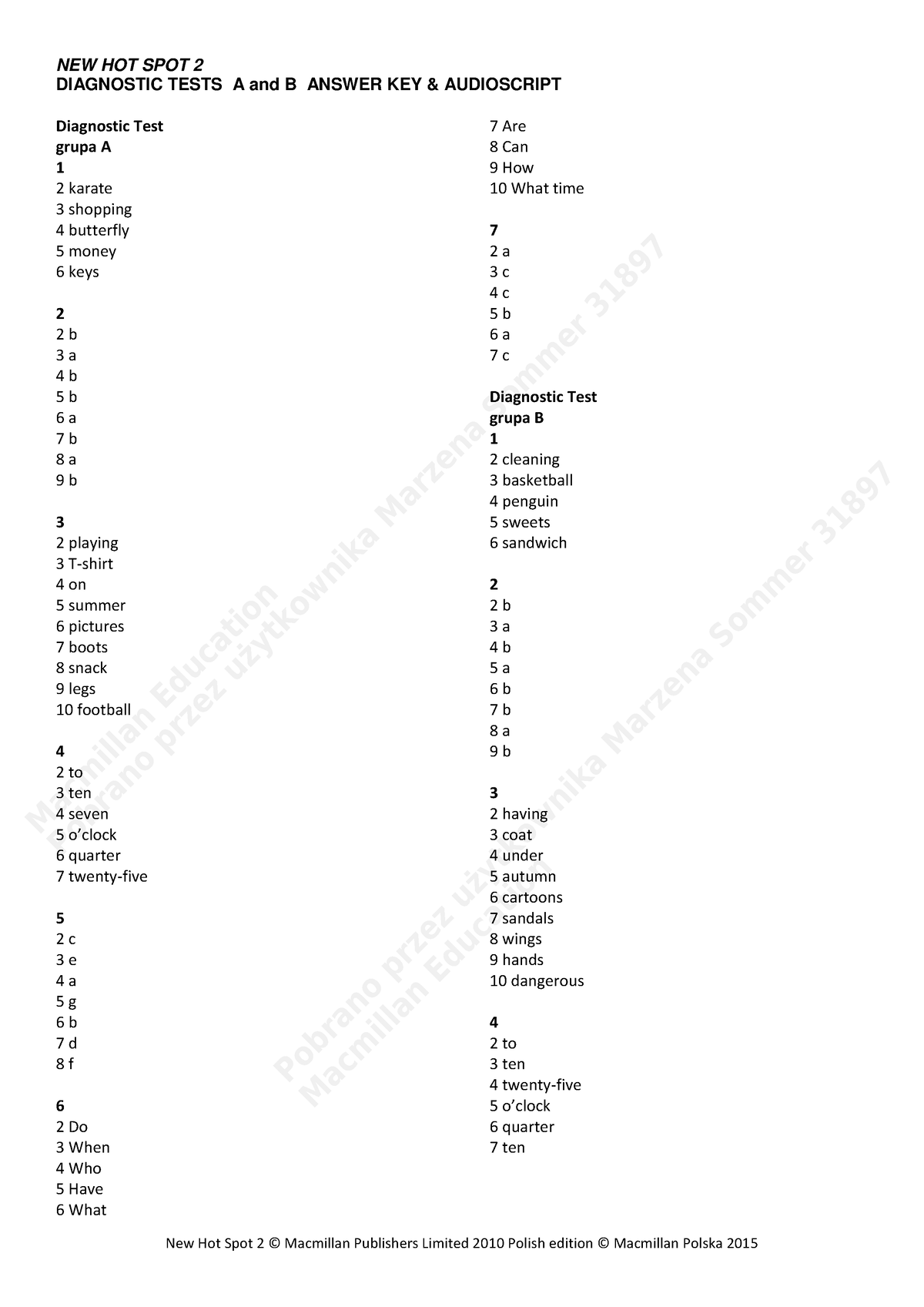The image features a white background with black text. At the top, in capital letters, it reads: "NEW HOTSPOT TO DIAGNOSTIC TEST A AND B ANSWER KEY AND AUDIO SCRIPT." Below, there is a list indicating various items associated with a diagnostic test. The list is as follows:

1. Blank 
2. Karate 
3. Shopping 
4. Butterfly 
5. Money 
6. Keys

Following this, the answers for Test A are provided: 
- 2: B 
- 3: A 
- 4: B 
- 5: B 
- 6: A 
- 7: B 
- 8: A 
- 9: B

Next, the answers for Test B are detailed: 
- 2: Plan
- 3: T-shirt 
- 4: On 
- 5: Summer 
- 6: Pictures 
- 7: Boots 
- 8: Snack 
- 9: Legs 
- 10: Football

Additionally, some miscellaneous answers are mentioned:
- 4: 2
- 2: 3
- 10: 4 
- 7: 5 o'clock 
- 6: Quarter
- 7: 25 
- 5: 2
- E